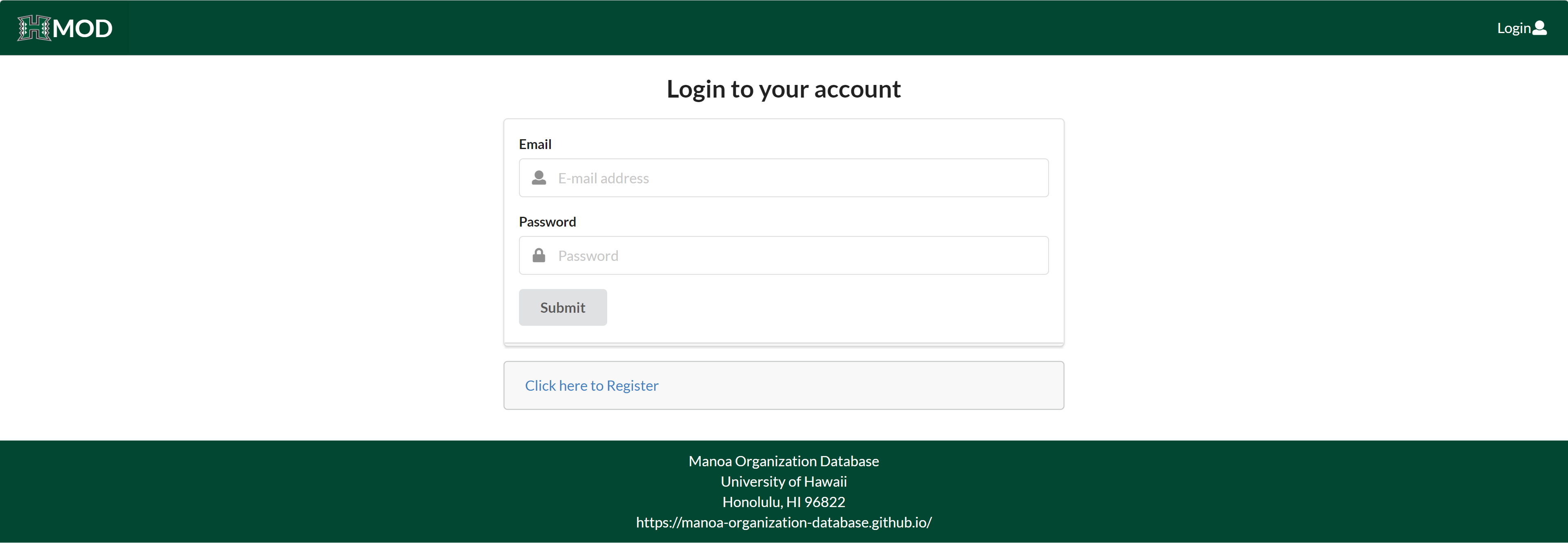This is a horizontally-oriented rectangular image depicting a webpage interface. At the very top of the screen, there is a horizontal hunter green bar stretching from the left to the right edge. On the left side of this bar, there is a small icon followed by the letters "MOD" in all capital letters. On the right side of this bar, the text "Log In" is displayed in white font, alongside a small image of a person.

Below this top bar, the center of the image features a large white rectangular section that occupies the majority of the page's width. In the middle of this section, the text "Log into your account" is displayed in black font. Underneath this heading, there are two input fields: one labeled "Email" and another labeled "Password," each with a blank space under their respective labels for user input. Following these input fields, there is a small light gray horizontal rectangular button labeled "Submit" in black font. Beneath this button, there is a line of turquoise text that reads "Click here to register."

At the bottom of the page, there is a thicker horizontal rectangular bar, larger than the top bar, also extending across the entire width. In the center of this bottom bar, there are several lines of very small white text. Although most of the text is difficult to read, it is clear that it includes the words "Honolulu, Hawaii" along with an area code, and a web address directly below that information.